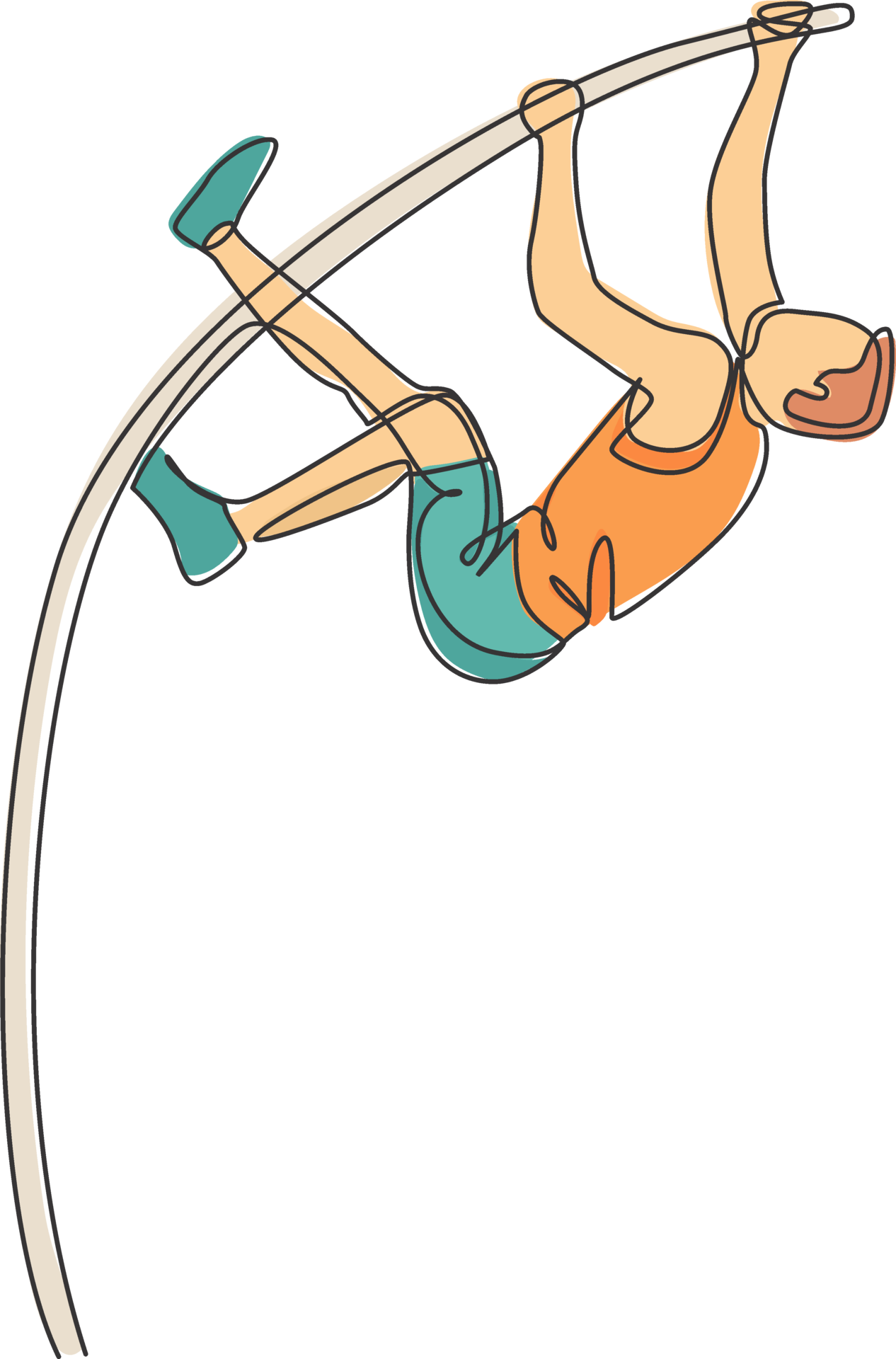The image is a detailed color drawing depicting a pole vaulter in mid-action, seemingly frozen at the peak of his vault. The background is a clean, solid white, providing no distractions from the athlete. The pole vaulter is a white man with short brown hair, wearing an orange sleeveless tank top, blue-green shorts, and matching blue-green shoes. His face lacks detailed features, emphasizing the motion over individual characteristics. The pole, which is light gray in color, is noticeably bent to the right. His right hand is gripping the top of the pole while his left hand is positioned just below it. His legs are dynamically posed, with one foot gripping the pole and the other extended outward. This image, resembling a watercolor painting, captures the essence and form of pole vaulting, focusing on the athletic prowess and technique involved in the sport.